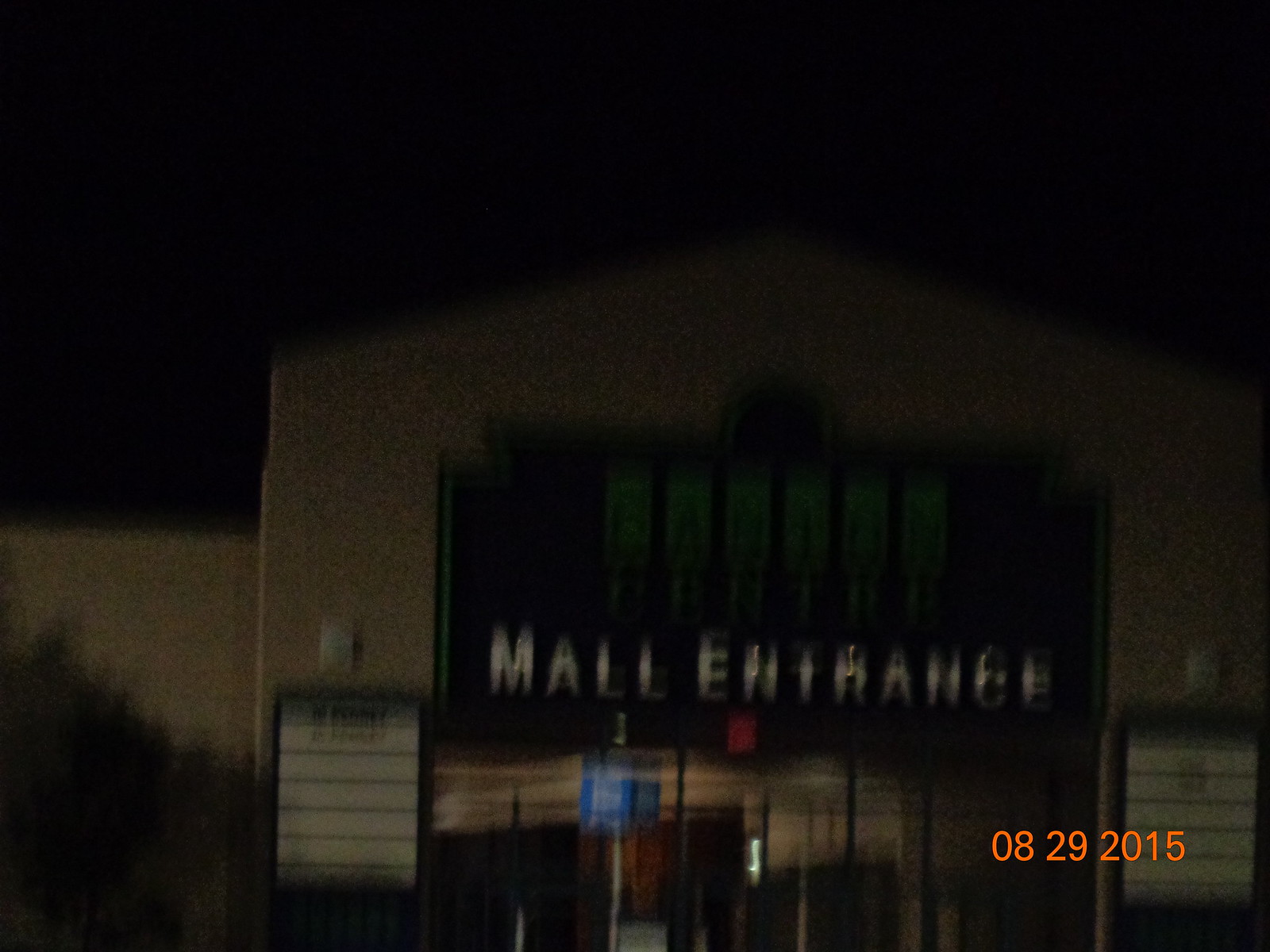In this very dark and blurry nighttime photograph, the sky is an impenetrable black, suggesting it was taken outdoors at night, specifically on August 29, 2015, as indicated by the date stamp in the bottom right corner. The main focus is an angled view of an entrance to a mall, with a brick facade that appears brown or stone-like. The entrance itself is notable for its pointed roof, which directs attention to a large black sign with a green outline. Centered on this sign, large green words are written, though they are not clearly legible. Beneath this, in smaller white text, the words "Mall Entrance" are distinctly visible. Adding to the scene's complexity, there is a blue sign in the foreground, resembling a bus stop, and a faint red glow beneath the "EN" in "Entrance," possibly from an exit sign. To the left of the entrance, the building features what looks like a movie marquee with a white background, and a similar marquee is on the right side, flanking the entrance. Additionally, a blurry image of a tree appears on the bottom left of the photo, partially obstructing the view of one of the white signs or windows on the side of the building. The array of colors in the image includes brown, white, green, black, blue, red, beige, and gray.